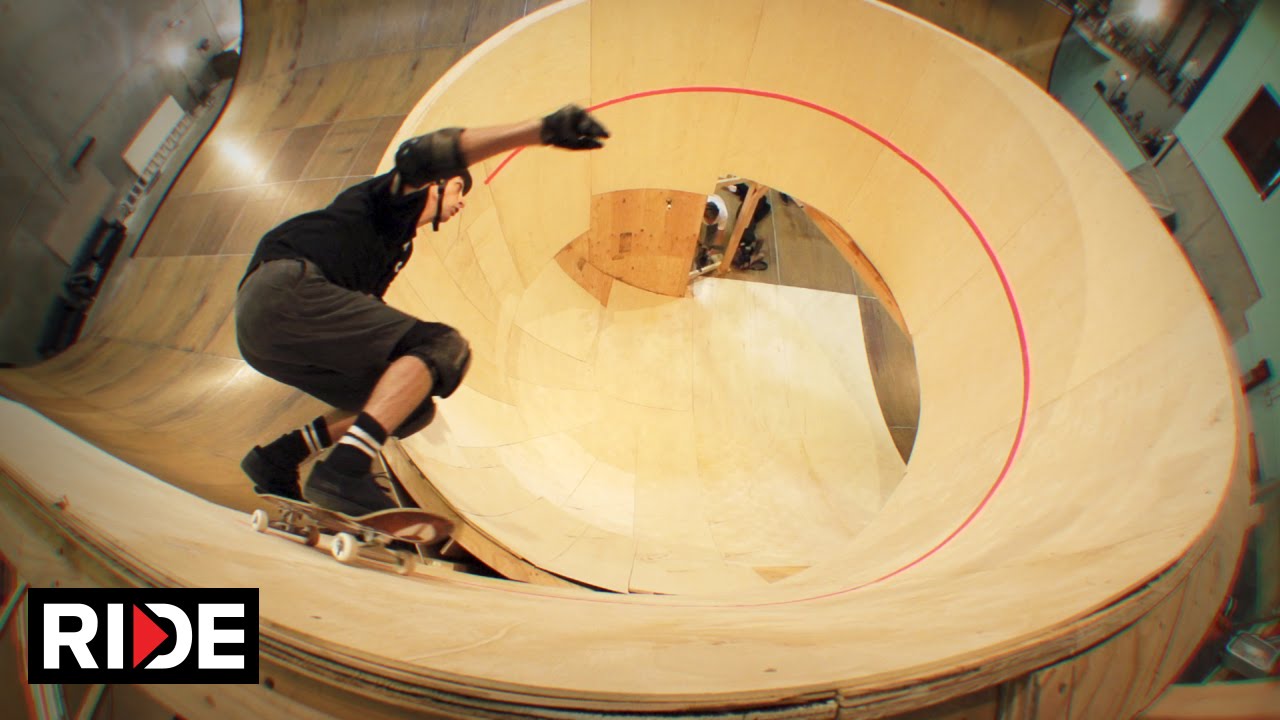The photograph captures a dynamic and artistic moment of a skateboarder navigating a complex skate park. The skateboarder, dressed in black with brown shorts, elbow, and knee pads, confidently rides a brown skateboard with a distinct wooden texture and a red line pattern. The skateboarder is positioned at the entrance of a spiraling, light beige wooden ramp that appears steep and challenging, suggesting a potential for danger if a fall occurs. Distinctively, the bottom left corner of the image features a black rectangle with the word "RIDE" in bold white letters, the letter D accented by a red triangle. The scene appears to be shot from an elevated angle, offering a comprehensive view of the spiral pipe-like structure that seamlessly transitions from a half-pipe setup, underscoring the skill required to navigate both the vertical and circular elements of the skate park.